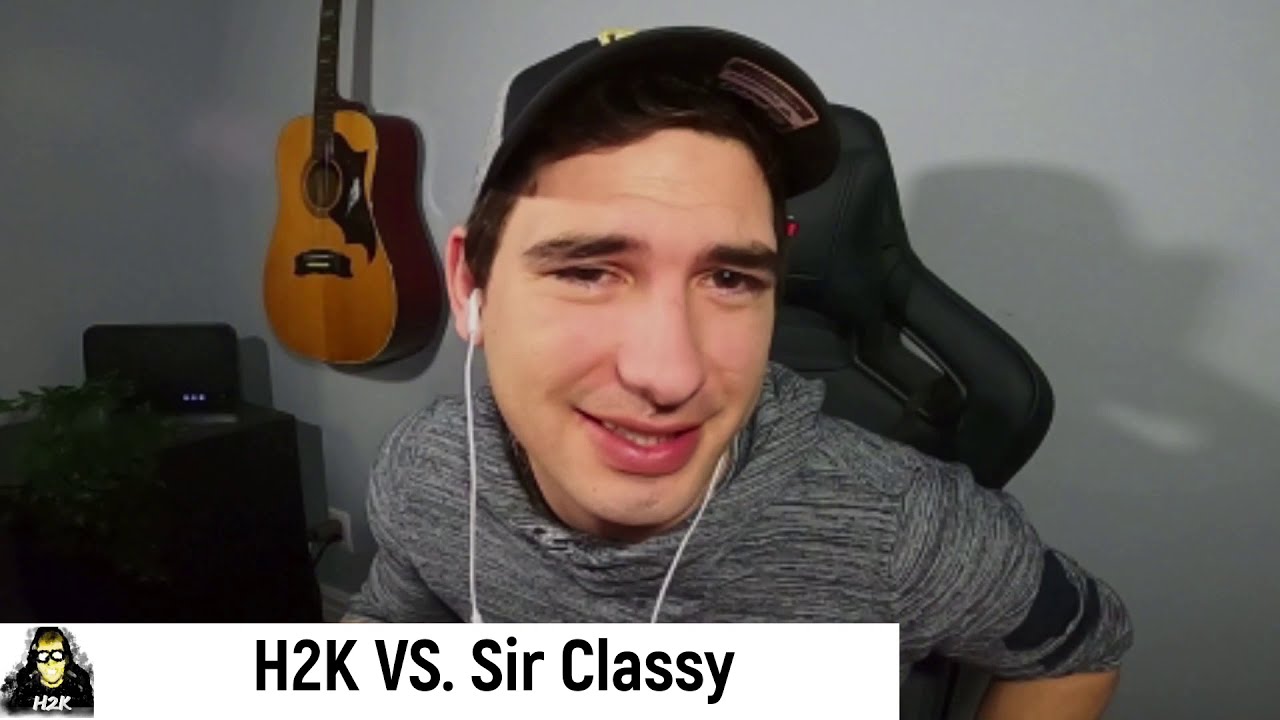The image shows a young Caucasian man, likely in his mid-20s, sitting directly in the center of the frame in a high-backed black gaming chair. He is wearing a black baseball cap with yellow text, a gray hoodie adorned with black horizontal stripes, and is listening through white wired earbuds. His expression is a confused smile as he looks slightly to his right. The backdrop is an indoor setting reminiscent of a YouTube video or Zoom call, featuring an off-white wall. On the left, a mahogany acoustic guitar hangs horizontally with a black speaker or amplifier below it. Additional details in the room include possible furniture and objects like a plant. Dominant colors in the image are white, black, tan, gray, pink, red, light brown, and green. A banner occupying about 10% of the image’s height runs along the bottom, and features a caricature of the person on the lower left. The text within the banner reads "H2K versus Sir Classy."